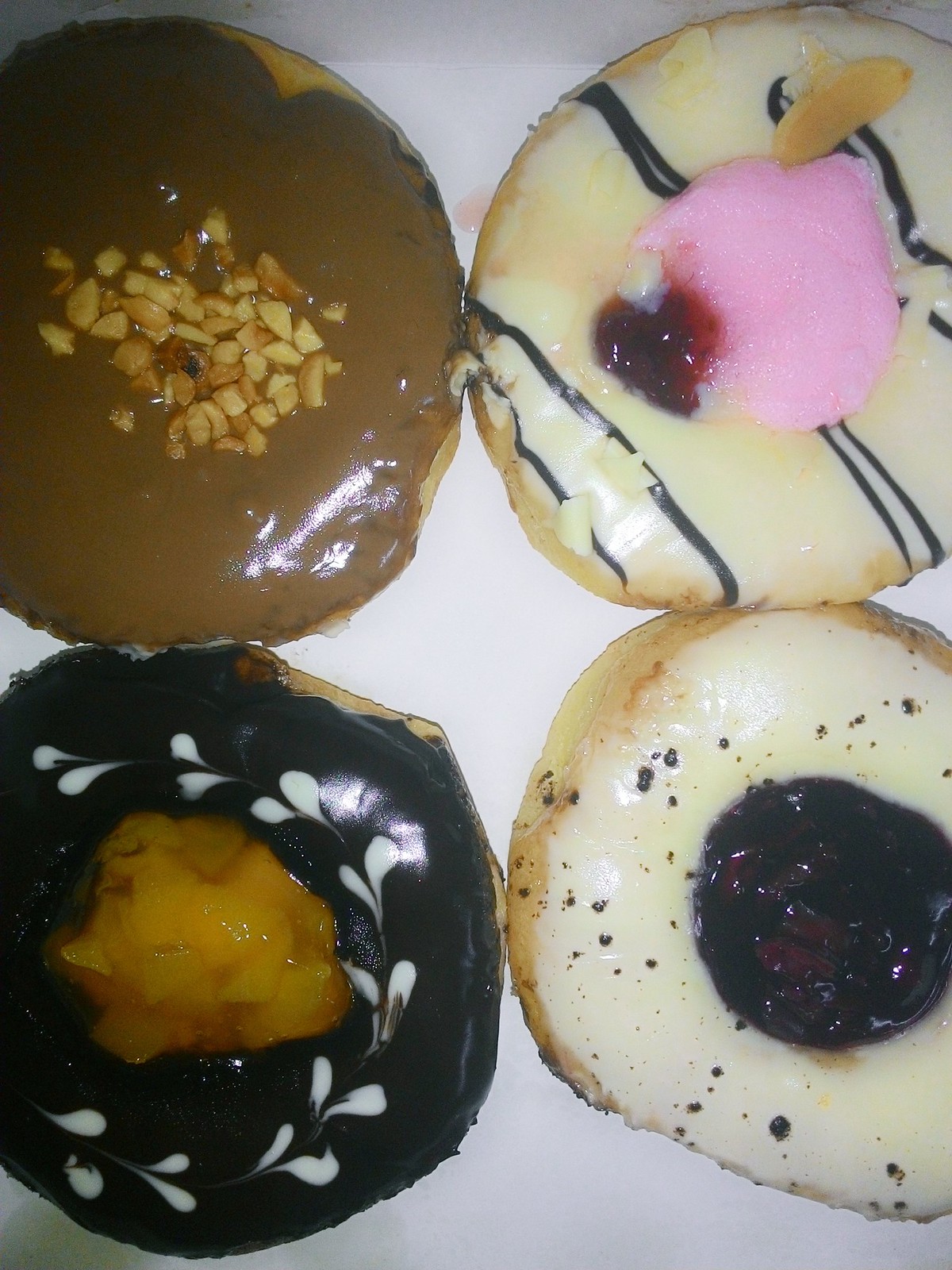This top-down photograph showcases four assorted donuts, arranged in a square on a dark background. The top left donut features a light brown icing, possibly maple-flavored, adorned with a sprinkle of chopped peanuts in the center. The top right donut has a white icing base embellished with vertical black stripes, encircling a pink center that could be strawberry-flavored, with a small jelly heart adjacent to the center. The bottom left donut is covered in a dark, nearly black icing, with a white floral pattern near the middle, which contains what looks like a peach filling. Lastly, the bottom right donut has a white icing scattered with black dots, and a central filling resembling blueberry jelly. The image is likely taken with a flash, highlighting the vibrant colors of the donuts while keeping the edges of the frame in relative darkness.